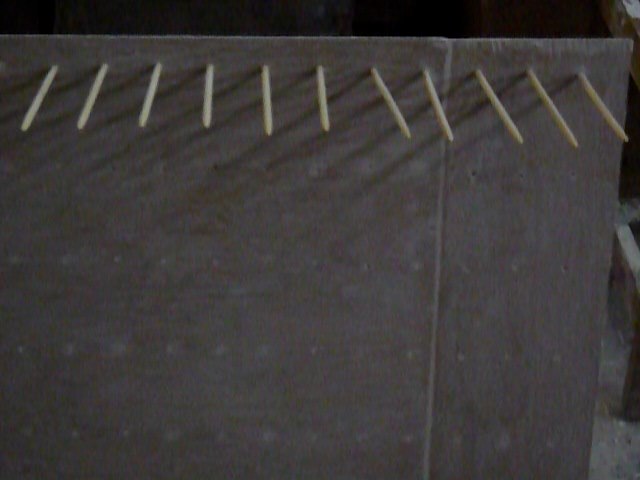The photograph is an indoor close-up of a heavy, well-worn brown cloth, which appears to cover or be attached to an unknown object, possibly a box. The cloth features a finished, rolled edge at the top with an opening, suggesting it might be a bag or container. Protruding from the upper portion of this cloth are 11 evenly spaced pegs or stakes that are tan to greenish-brown in color, appearing either as nails or wooden sticks. They are pointed and project outward towards the camera. The light source is coming from the upper right, casting shadows diagonally to the lower left, which adds depth to the image. The background and the majority of the photograph is in dark, muted tones, with shades of gray and black, giving the overall image a slightly out-of-focus and dull appearance.